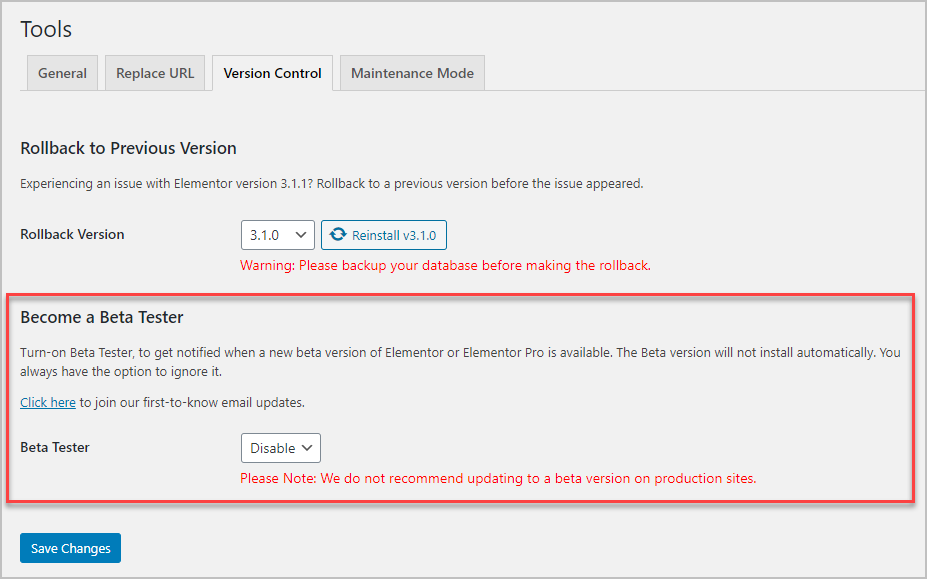This is a detailed and descriptive caption for the provided screenshot:

The screenshot features a computer interface with a gray background in the upper left corner. At the top, in black text, it says "Tools." Two lines below this, there are four tab-like boxes labeled "General," "Replace URL," "Version Control" (which is bolded), and "Maintenance Mode." 

Approximately four to five lines down, on the left side, bolded in black text, it reads "Rollback to Previous Version." Two lines below, in black, it says, "Experiencing an issue with Elementor version 3.1.1? Rollback to a previous version before the issue appeared." 

Three lines down from this text, on the left side, it says "Rollback Version" in black. Slightly to the right of this, there is a white box with gray text inside that reads "3.1.0," accompanied by an upside-down "V" symbol. To the right of this box, there is a rectangle outlined in blue, featuring a blue circle on the left and the text "Reinstall v3.1.0" in blue to the right of the circle. 

Beneath these elements, in red text, it warns, "Warning: Please backup your database before making the rollback." Two lines below this warning, there is a rectangle outlined in bold red. In the upper left-hand corner of this rectangle, in black, it says "Become a Beta Tester." 

Two lines underneath, in black text, it says, "Turn-on Beta Tester to get notified when a new beta version of Elementor or Elementor Pro is available. The beta version will not install automatically. You will always have the option to ignore that." 

The phrase "Click here" is in blue and underlined, suggesting a hyperlink, followed by "to join our first-to-know email updates." 

Three lines below this, in bold black text, it says "Beta Tester." To the right of this, there is a rectangle outlined in gray with the text "Disable" in black inside it, alongside a downward-pointing "V" symbol. 

Underneath this box, in red text, it states, "Please note: We do not recommend updating to a beta version on production sites." 

In the lower left-hand corner, there is a blue rectangle with the text "Save Changes" in white inside it.